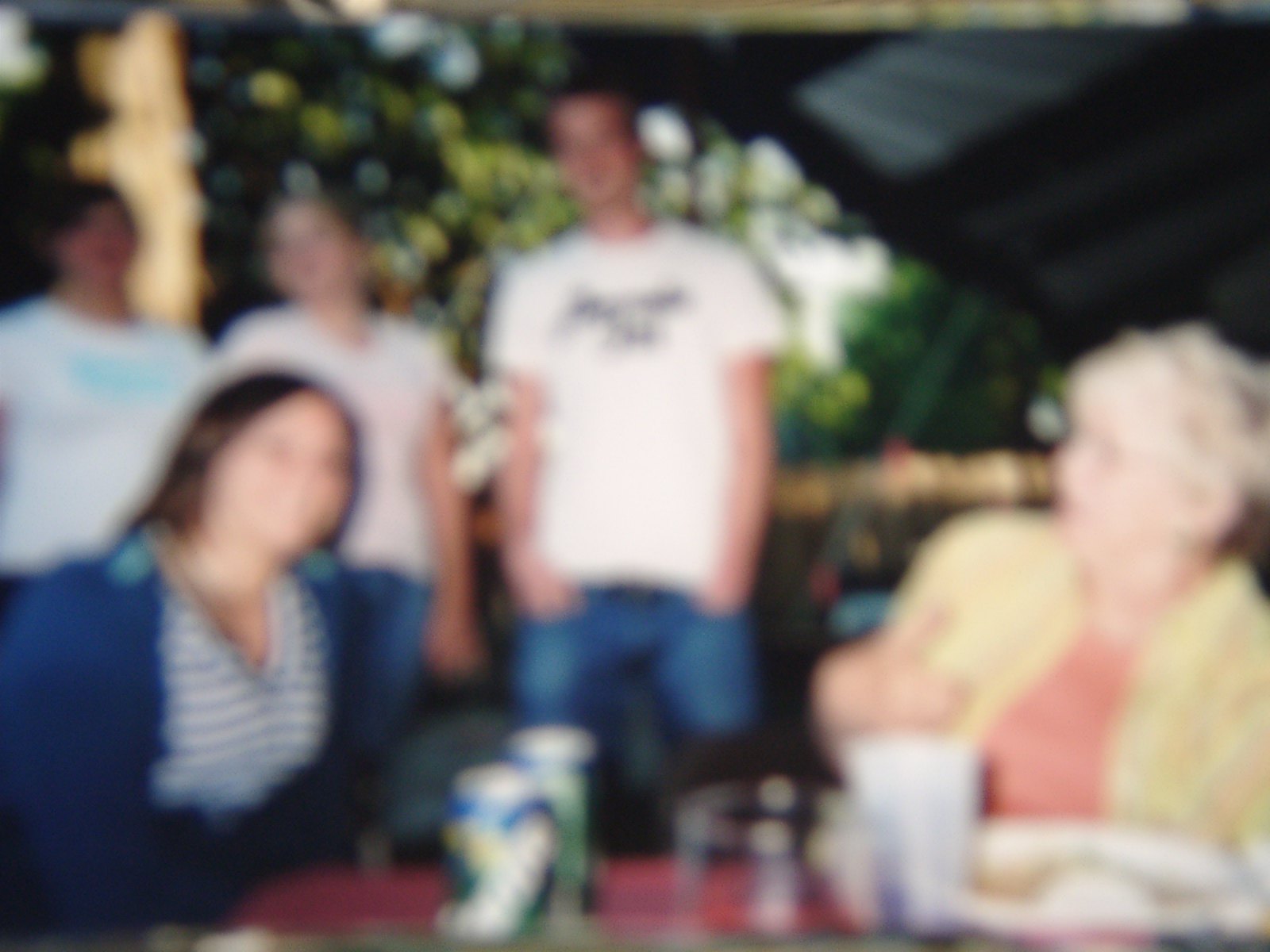The photograph captures a group of five individuals in an outdoor setting, likely a porch, deck, or backyard area with some trees visible in the background. The image is notably blurry, making it difficult to discern fine details or facial expressions clearly. In the foreground, two women are seated at a table adorned with a few soda cans, possibly Sprite, and additional cups. The younger woman on the left wears a blue and white-striped shirt and is smiling at the camera, her features indistinct due to the photo’s poor focus. Next to her, the older woman on the right, dressed in a beige coat with a tan or orange shirt, appears to be reacting with surprise or shock to something the younger woman is saying. Standing behind them are three younger individuals, likely teenagers or young adults, all clad in white shirts and blue denim jeans. The group is enveloped by a camping-like black mesh screen, with dappled sunlight filtering in from the left. Despite the blurriness, the photograph conveys a casual, joyous moment shared among family or friends in a relaxed outdoor environment.